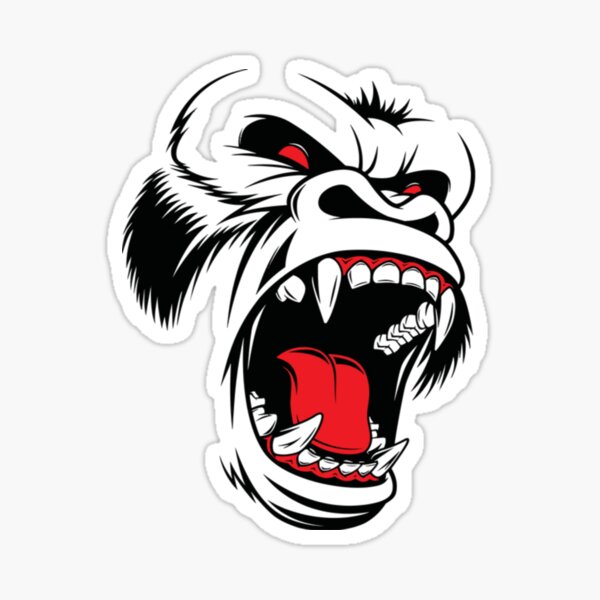The image features a striking sticker of a gorilla's face, rendered with a dramatic and intense color palette of black, white, and red. The gorilla's predominantly black face is accentuated with bold outlines, highlighting its fierce expression. Its eyes are particularly menacing, glowing red and adding to the overall aggressive demeanor. The open mouth reveals menacing white fangs – two on the upper jaw and two on the lower – while the rest of its teeth are white and flat, framed by vivid red gums and a protruding red tongue that heightens the intensity of the image.

Long, detailed fur adorns the sides of its cheeks, adding texture and depth to the illustration. Between its piercing red eyes lies a small tuft of black fur, further emphasizing its menacing gaze. The gorilla's face is completed with thick, pronounced eyebrows and a large, wide nose, both adding to its fearsome appearance. The entire sticker is set against a solid gray background, which serves to bring the vivid and detailed elements of the gorilla's face into even sharper relief.